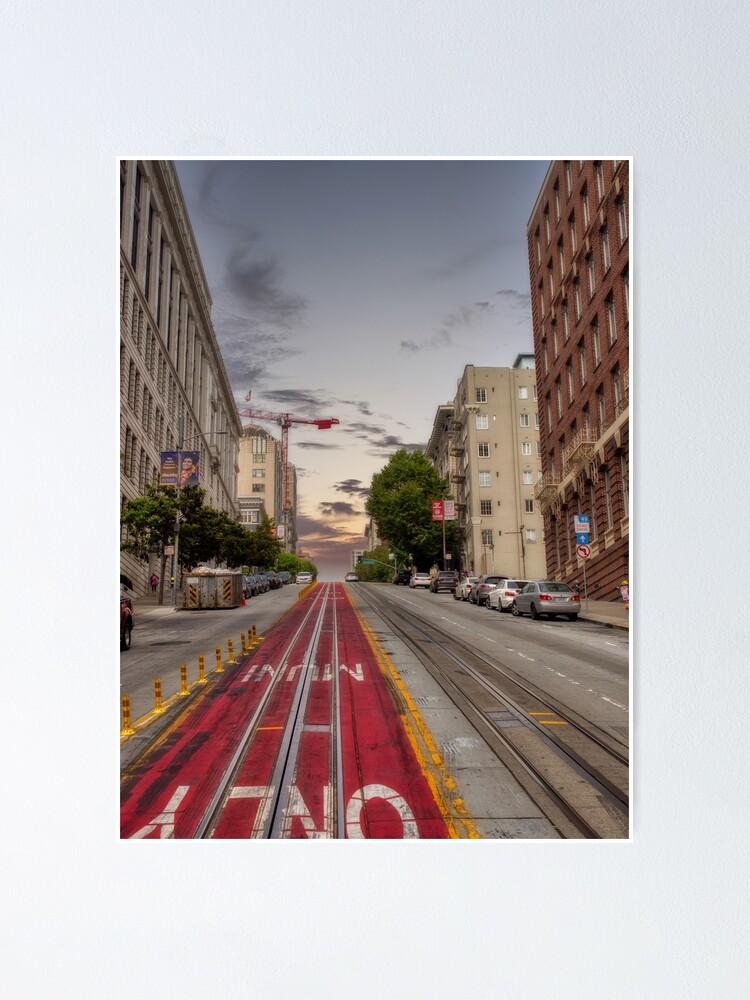The image depicts a bustling city street, likely in San Francisco, characterized by its hilly terrain and iconic cable car tracks running up the middle. We're positioned in the middle of a red-painted lane with yellow stripes, designated "Muni Only" for exclusive cable car use, the white lettering noticeably backward from our vantage point. The street is lined with intermittent black and white poles, and several red or orange striped posts. Cars are parked along both sides of the street, which slopes steeply uphill, their parking brakes presumably set.

Dominating the scene are several tall buildings, including a prominent cream-colored structure to the left and a red brick building to the right, both flanked by additional multistory edifices further up the hill. The sidewalks are adorned with green trees, adding a touch of nature to the urban landscape.

Above, the sky transitions from a bright blue to hues of orange and gray, suggesting either a sunrise or sunset. The scene is also marked by the presence of a mechanical crane in the distance, indicative of ongoing construction or development in the area. The overall atmosphere captures the dynamic and evolving essence of a classic San Francisco street.